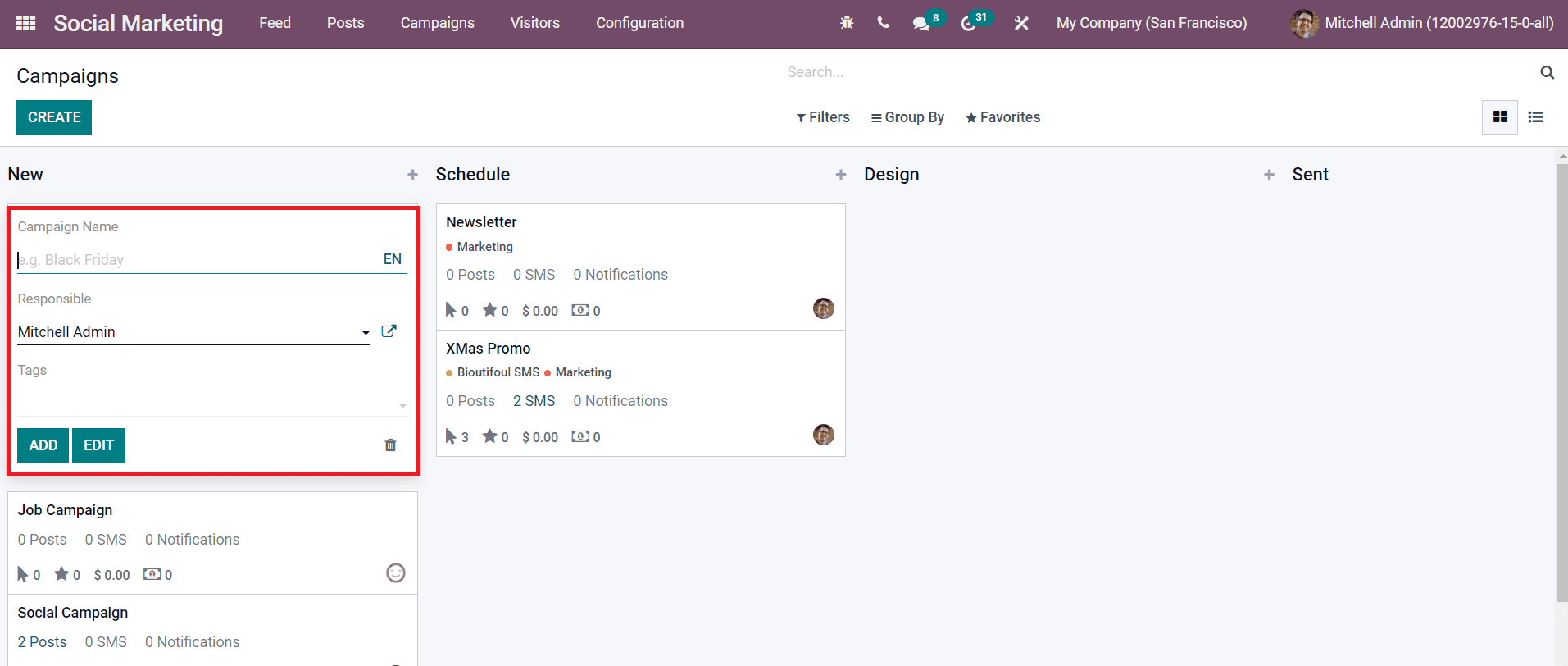A screenshot of a marketing program interface is displayed, likely from a company in San Francisco, though the specific website is not identified due to the absence of a browser bar. The top section features a prominent purple bar labeled "Social Marketing" on the left, with menu options including "Feed," "Post," "Campaigns," "Visitors," and "Configuration" to its right. 

Below this main menu, on the left-hand side, there's a sidebar with a "Campaigns" header and a blue "Create" button beneath it. Adjacent to the "Create" button area is a search bar where users can type in queries. Underneath the search bar, options for "Filters," "Group By," and "Favorites" are available.

In the "Campaigns" section, there is a detailed form titled "New," which allows the creation of new campaigns by entering a campaign name and assigning responsibilities. Below this form, users can find buttons for "Add" or "Edit." To the right, there is a section dedicated to scheduling, with options to schedule newsletters, marketing campaigns, and Christmas promotions.

Further to the right are additional sections for "Design" and "Send," but both sections currently offer no available options. The "New" campaign form also includes additional options for specifying the type of campaign, such as "Job Campaign" and "Social Campaign." The program's administrator is identified as Mitchell.